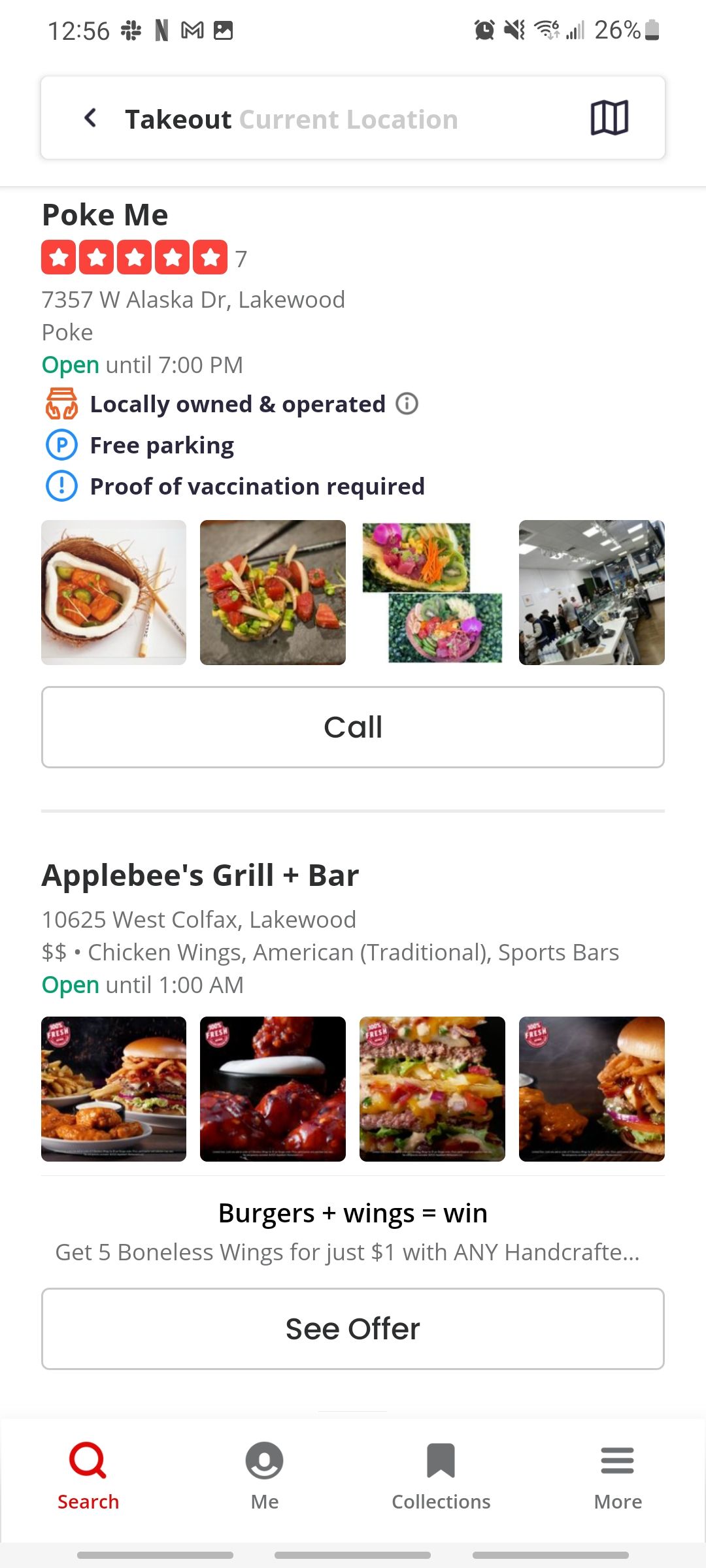This image captures a screenshot of a mobile device's home screen. In the top left corner, the time is displayed as 12:56 PM. Notifications from various apps, including Netflix, the Gmail app, and the gallery, are visible. On the top right, there are icons indicating an alarm notification, the device being on mute or vibration mode, the cellular network signal strength, and a battery level at 26%. Below, there is a banner featuring information about a local Applebee's Grill and Bar. The banner highlights that the establishment is locally owned and operated, offers free parking, and requires proof of vaccination. Additionally, it features the tagline "Hook Me" and touts a rating of 5 stars out of 7 based on customer reviews.